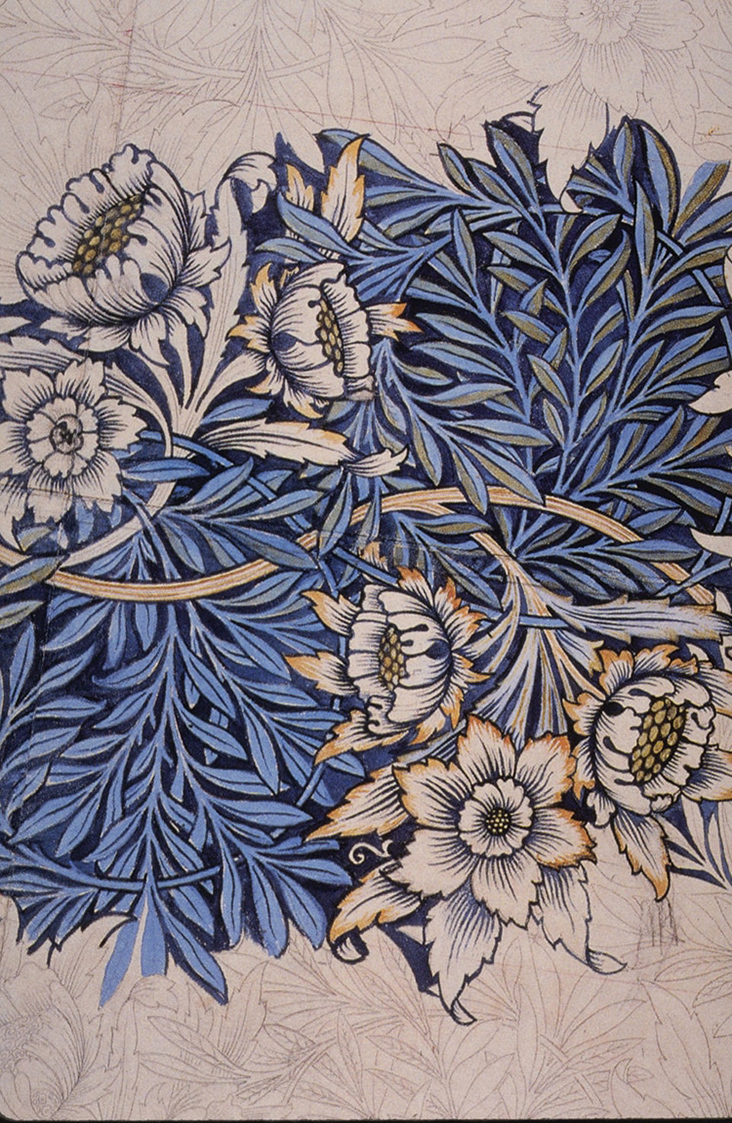This intricate painting showcases an elaborate and detailed flowery pattern set against a tan background adorned with etched vines and flowers. The central focus is a collection of leaves rendered in varying shades of blue and moss green, which interweave throughout the composition, stretching from the upper left corner to the lower right corner. The flowers, meticulously drawn in black pen, possess petals that match the beige color of the background, with some edges tinged in orange. The centers of these blossoms are highlighted with vibrant yellow circles encased in a black border. Despite its intricate details, this piece maintains a subdued color palette, with the petals largely appearing white with black streaks and occasionally accented with blue. This artwork, possibly appearing as a tiled design, flooring, tablecloth, or even clothing fabric, captures an essence of nature through its flowery motifs and textured, sketched elements, although the exact medium or application remains undetermined.